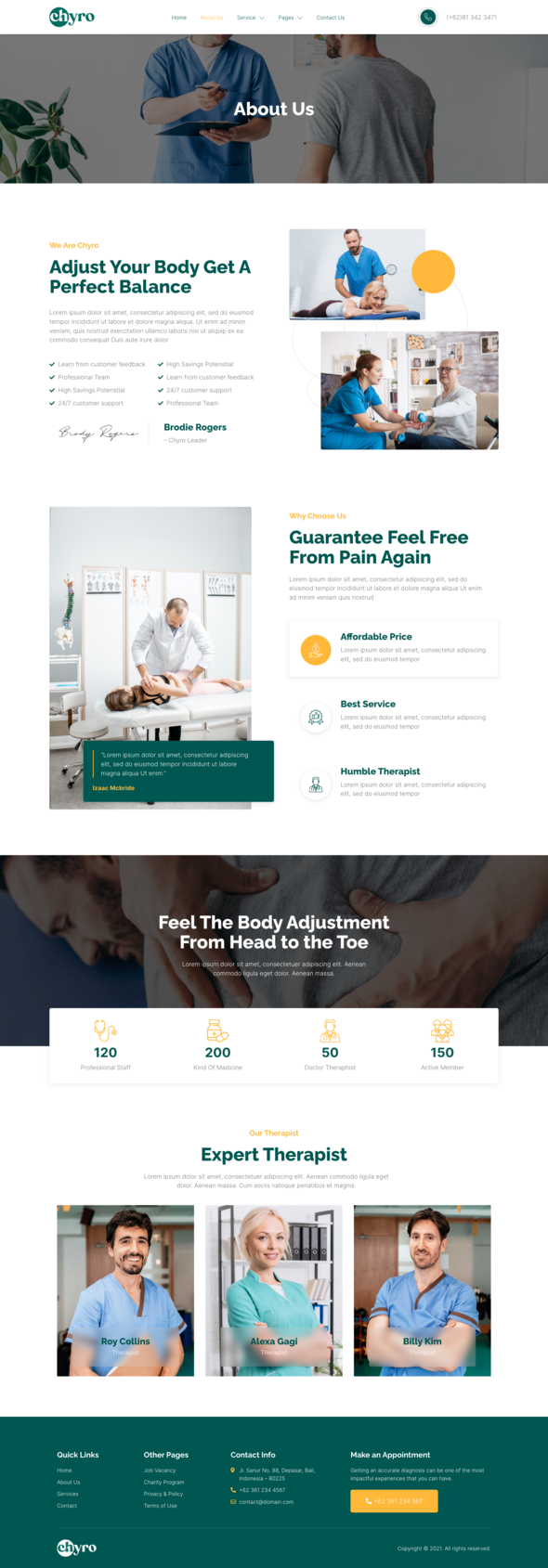This image is a detailed screenshot of the "About Us" webpage for a company called CH Pro. The company’s logo, featuring "CH" in white text encircled by green and followed by "PRO" in green text, is prominently displayed in the upper left-hand corner of the page.

At the top center of the image, small links seemingly direct users to different sections within the website, though the text is too small to be legible.

Centered below these links is a rectangular photograph showing two individuals from the waist up to their neck. The person on the left faces the camera, while the individual on the right has their back turned. Situated beneath the photograph, large text reads "About Us."

The main content area is divided into several sections with blurbs and additional visuals. The first blurb, located in the upper left part of the content area, reads "Adjust your body to get a perfect balance," accompanied by smaller, unreadable text and images to the right.

Further down, there is an image on the left side depicting a person either receiving a massage or a chiropractic adjustment. Adjacent to this image, another section of text states "Guarantee feel free from pain again," and includes clickable links.

The bottom part of the content area has a section with the heading "Feel the body adjust from head to toe," followed by more text that is too small to discern. Additionally, this section prominently features the profiles of three expert therapists – two men and one woman, providing a conclusion to the visual layout of the webpage.